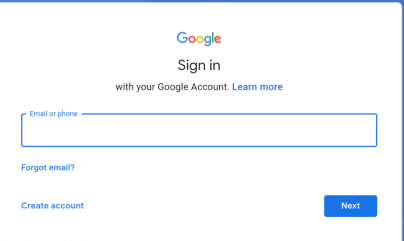The screenshot captures most of the Google sign-in page, slightly cropped on the left and bottom edges. A thin blue line runs horizontally along the top edge, while another thin blue line runs vertically down the right side. No lines are present on the left or bottom edges. 

At the top center of the page is the Google logo, with "Google" displayed in its iconic font and colors: blue, red, yellow, and green. Below the logo, the text reads, "Sign in with your Google account." There is a "Learn more" link in blue text beneath this introduction.

A wide, rectangular, vertically oriented input box for entering an email address or phone number is positioned below. Directly under the input box, options are provided for users who may have forgotten their email or wish to create a new account. 

In the bottom right corner of the screenshot, there is a blue rectangular button labeled "Next."